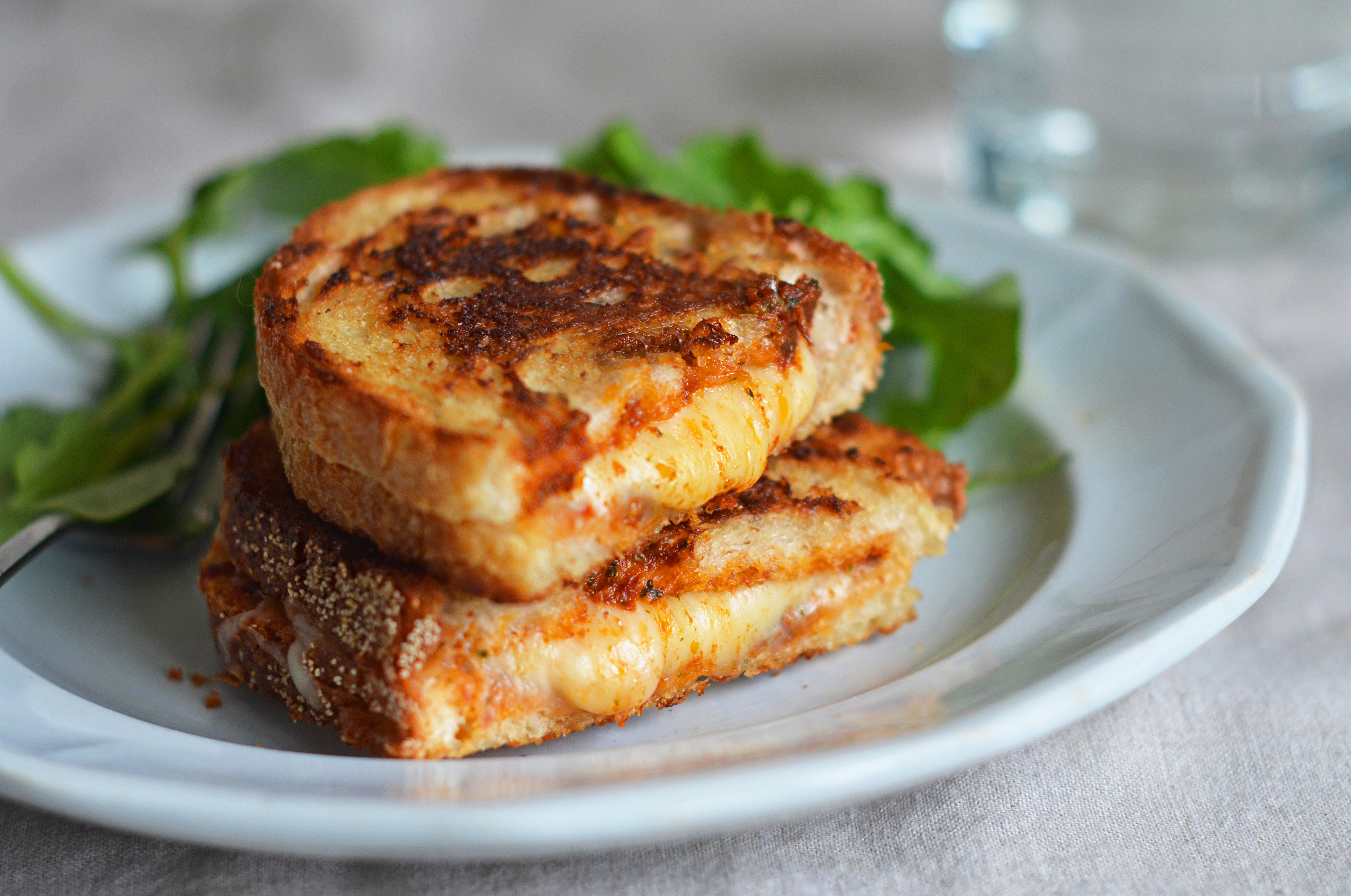This close-up photograph depicts a mouthwatering grilled cheese sandwich, cut in half and stacked atop each other on a reflective white porcelain plate. The sandwich features golden brown sourdough bread, perfectly toasted, with gooey yellow cheese oozing out from the middle. The sandwich is set against a white tablecloth, with a bed of fresh arugula leaves and a fork positioned behind it, adding a touch of green and a side garnish to the composition. Notably, the left side of the grilled cheese showcases white grains on the bread’s edge and some crumbs scattered on the plate. The background of the image is blurred, with an out-of-focus clear glass in the top right, adding depth to the photo. The overall scene is inviting and emphasizes the textures and colors of the delicious sandwich.